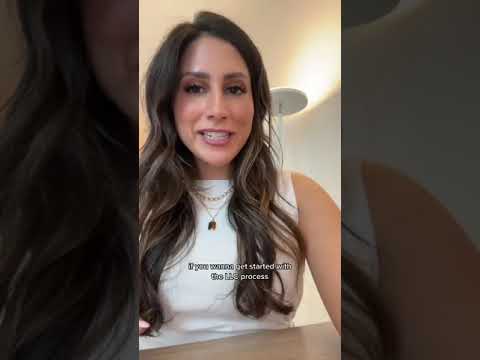In the image, a young woman, possibly in her late 20s or early 30s, is sitting indoors, perhaps in a bedroom or dining room. The setting includes light yellow walls and a white ceiling, with a tall lamp in the background casting a warm glow on the ceiling. The scene appears to be captured from a cell phone, reminiscent of content typically seen on TikTok or Instagram.

The focal point is the woman, who is smiling and looking directly at the camera as if speaking to her audience. She has long, slightly curly brown hair that flows past her shoulders and has a well-made-up face with particularly long eyelashes and emphasis on her cheeks. She wears a white tank top and three delicate necklaces, one of which features an indistinguishable charm. 

In front of her is a light wooden table. Superimposed on the lower portion of the image is small white text that reads, "if you wanna get started with the LLE process," suggesting a promotional or instructional context, potentially pitching a service or program referred to as 'LLE.'